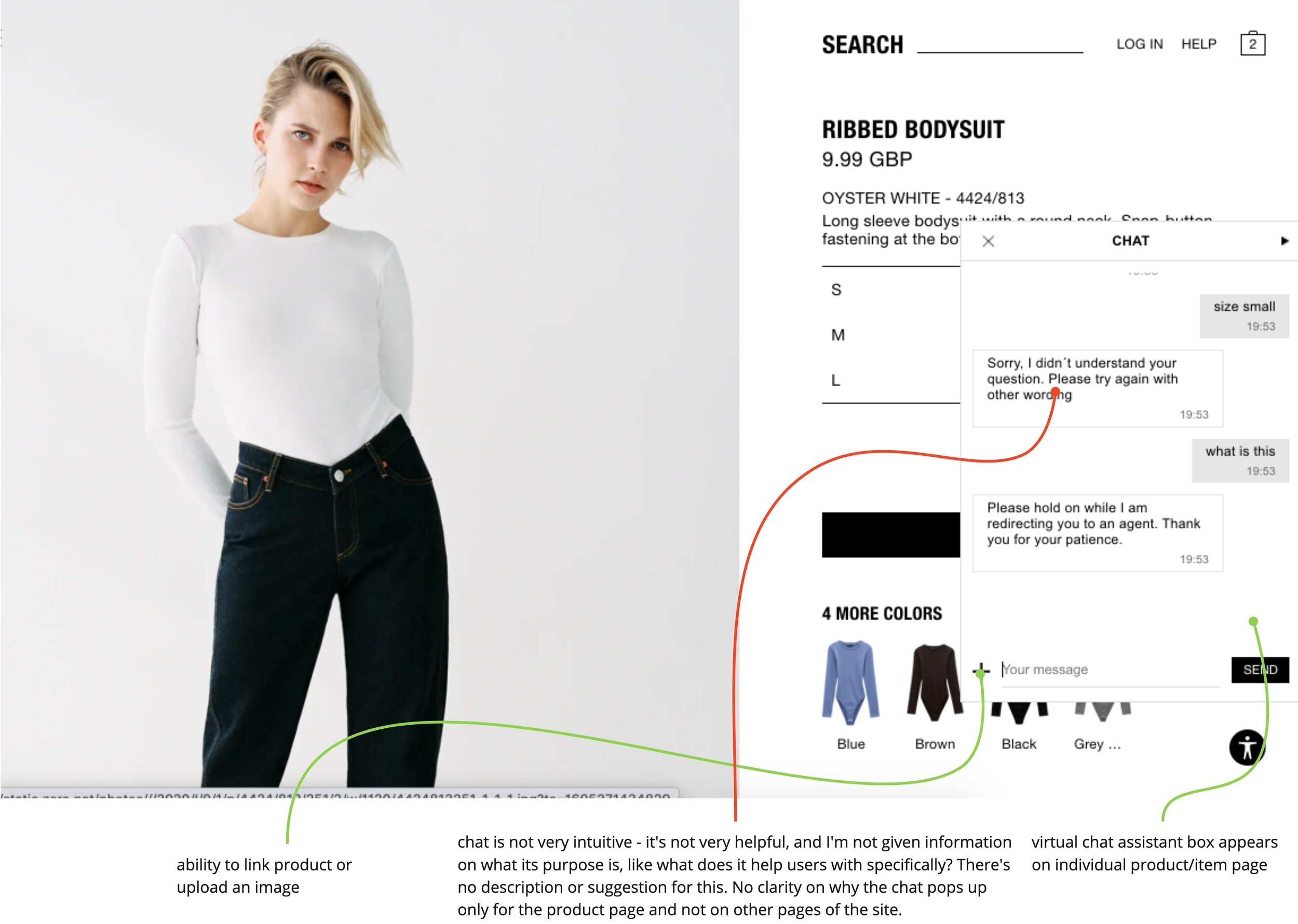The image is a horizontally-oriented rectangle, reminiscent of a screenshot from an online shopping website. On the left side, a promotional photo features a woman with fair skin and red lipstick. She stands with her arms behind her back and gazes directly into the camera. She is wearing a form-fitting, long-sleeved, white ribbed bodysuit paired with black jeans. Her semi-short hair frames her face, and the backdrop encompasses a pristine white setting, keeping the focus on the product.

Moving to the right portion of the image, the layout includes a search bar at the top alongside options for login and help. Below, the product details are succinctly stated: the item is a "Ribbed Bodysuit" priced at 9.99 GBP in an "Oyster White" color. The product description is partially obscured by an active chat window overlay.

The chat interaction involves automated customer support, responding initially with, "Sorry, I didn't understand your question. Please try again with other wording." The customer queries, "What is this?" leading the chat system to reply, "Please hold on while I redirect you to an agent. Thank you for your patience." Various arrows and a green line are present, seemingly part of a feature explanation. One arrow points to the chat window, highlighting the "ability to link product or upload an image."